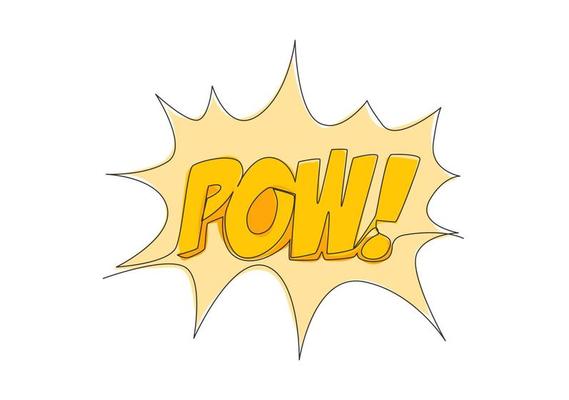A striking comic book stylized image featuring a dynamic, jagged-edged sound bubble dominates the scene, set against a clean, background-free canvas. The interior of the sound bubble is filled with a vibrant light yellow hue, while the center prominently displays the bold, capitalized text "POW!" in dark yellow. The powerful word is meticulously outlined, creating a seamless integration between the interior and exterior with a continuous solid line. Adding to the dramatic effect, the "POW!" text is accentuated by subtle, darker yellow shading, giving the image depth and an explosive, three-dimensional appearance.